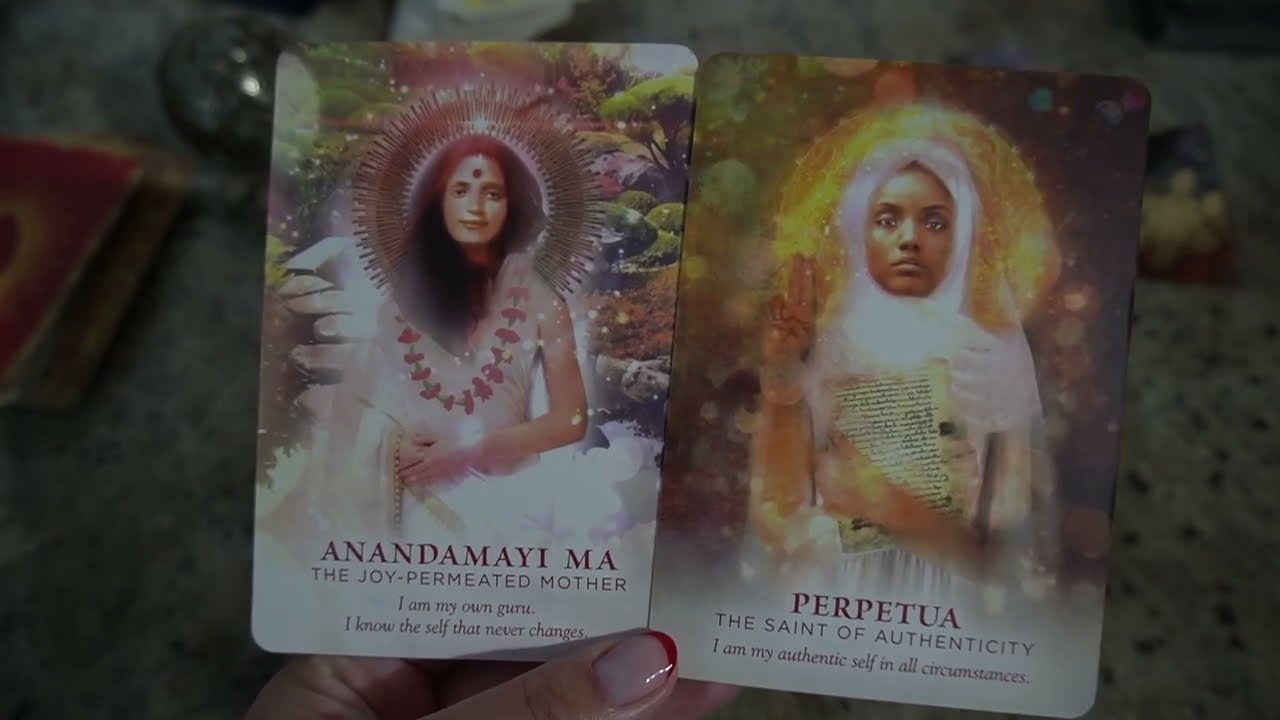In this detailed rectangular image resembling a postcard, the blurred background hints at a countertop with scattered cards. Dominating the foreground are a woman's beautifully manicured left hand and glossy fingernails, adorned with light pink or white polish and red-tipped nails. Her thumb and fingers prominently hold up two intricate cards side by side.

The left card features a Croatian woman with long, dyed red-brown hair flowing beneath an elaborate peacock-like headdress. Adorned in a white top with a garland of red flowers, she embodies serenity. The text on her card reads, "Anandamayi Ma, the joy-permeated mother," accompanied by "I am my own guru, I know the self that never changes." Some details like beads are also present on this card.

The right card presents a solemn black woman with caramel-colored skin, framed by a golden aura and a white headdress. Her stern expression is both striking and profound. She dons a white top and holds an off-white page to her chest. Her card declares, "Perpetua, the saint of authenticity," with the message, "I am my authentic self in all circumstances." The imagery and text suggest these cards are tools for personal introspection and peace.